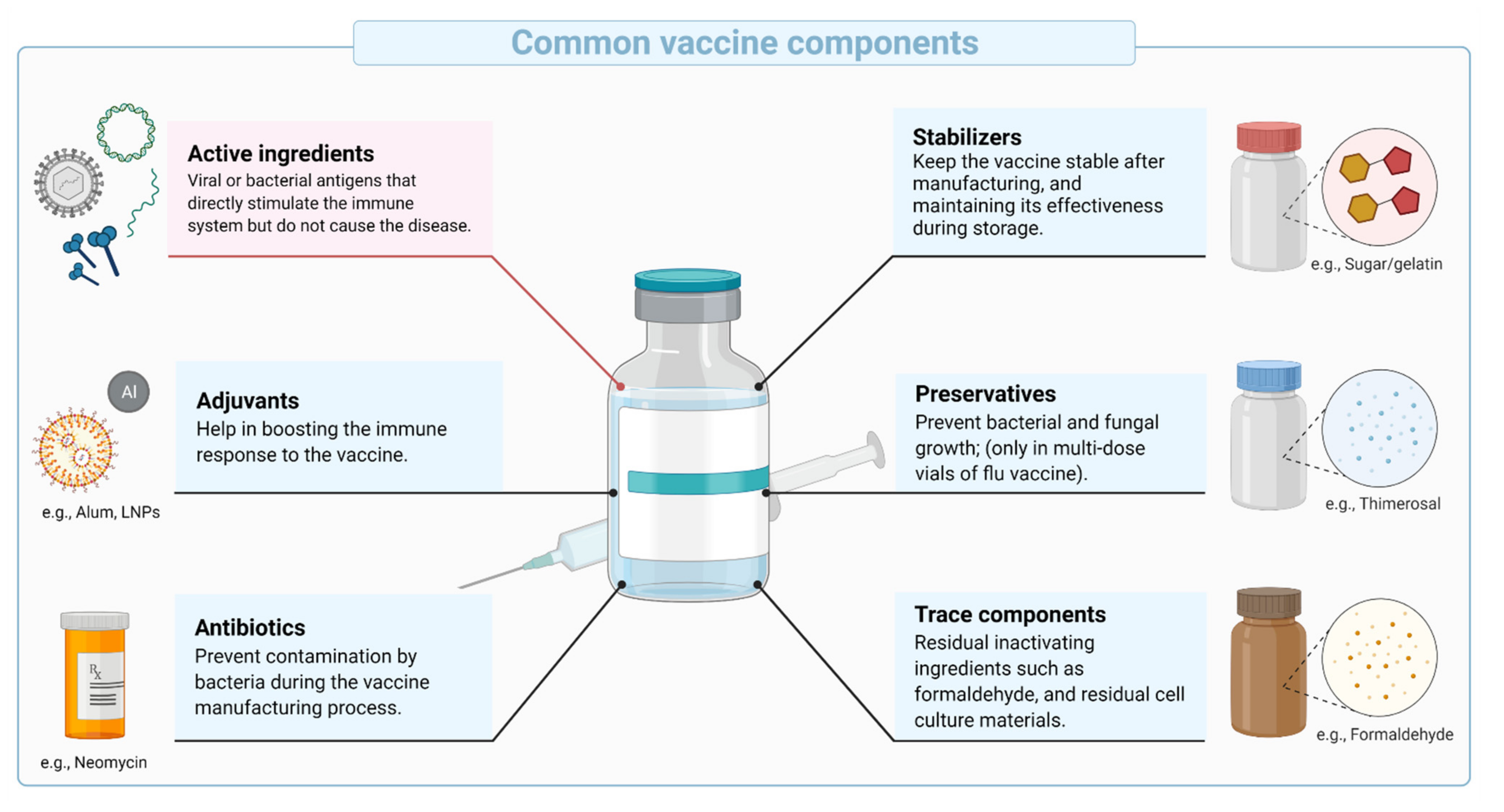This is a detailed illustrated diagram showing common vaccine components against a white background. Central to the image is a drawing of a blue and white medical vial in front of a syringe, with six lines connected to it, each leading to a box of text with small illustrations. The diagram’s title reads "Common Vaccine Components."

1. **Active Ingredients (Upper Left)**: Viral or bacterial antigens that directly stimulate the immune system without causing the disease. There are drawings of viruses and bacteria alongside this description.
2. **Adjuvants (Middle Left)**: Substances that help to boost the immune response to the vaccine. The illustration includes a circle labeled "Al" and a sun-like icon with examples such as Alum and LPNs.
3. **Antibiotics (Bottom Left)**: Used to prevent contamination by bacteria during the vaccine manufacturing process. The box contains a prescription bottle labeled “Example: neomycin.”
4. **Stabilizers (Upper Right)**: Keep the vaccine stable after manufacturing and maintain its effectiveness during storage. The visual includes a bottle with a red cap and a diagram of yellow hexagons and red pentagons, with examples like sugar and gelatin.
5. **Preservatives (Middle Right)**: Prevent bacterial and fungal growth in multi-dose vials, specifically for flu vaccines. This section shows a bottle with a blue cap and blue dots, with an example labeled “thimerosal.”
6. **Trace Components (Bottom Right)**: Residual inactivating ingredients such as formaldehyde and residual cell culture materials left from the manufacturing process. The visual here includes a brown bottle with a brown cap labeled with “Example: formaldehyde.” 

Each component is effectively illustrated with visual aids, providing a comprehensive understanding of the common elements found in vaccines.